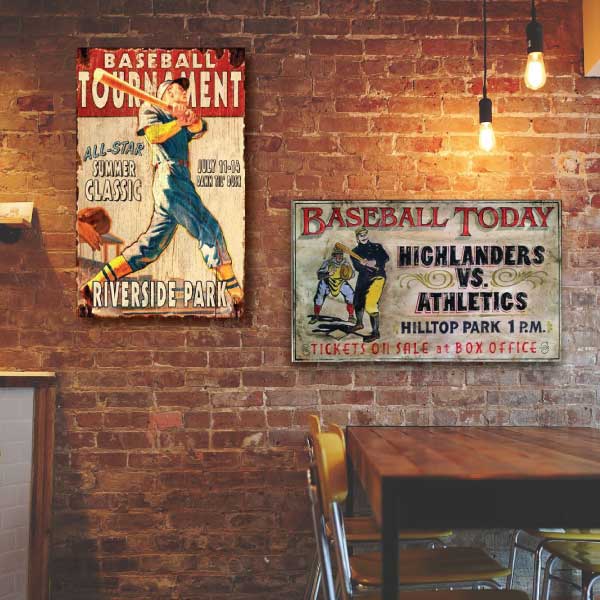The photograph captures a cozy corner of a restaurant, distinguished by its rustic red brick walls adorned with vintage metal signs and eclectic décor. The overall shape of the photograph is rectangular, with the left and right sides being marginally longer than the top and bottom. Dominating the upper portion of the image are two metal printed signs. 

On the left side, a rectangular sign proudly displays "Baseball Tournament All-Star Summer Classic, July 11th to 14th, Dawn at the Dome" with a vibrant illustration of a man in a blue and yellow uniform swinging a bat, the bat extending from the upper left towards the right. Adjacent to this, on the right side, another metal sign, rectangular in shape but oriented differently, reads "Baseball Today, Highlanders vs. Athletics, Hilltop Park, 1 p.m., tickets on sale at Box Office," accompanied by an image of two baseball players in action.

The setting includes a built-in table at the bottom right corner, seamlessly integrated into the red brick wall, surrounded by four chairs with yellow seat cushions and backs. A counter framed with wood and painted white bricks is visible in the bottom left, adding to the charm of the space. Overhead, in the top right corner, two fluorescent light bulbs hang from the ceiling, suspended by black wires, enhancing the warm, inviting ambiance of the restaurant.